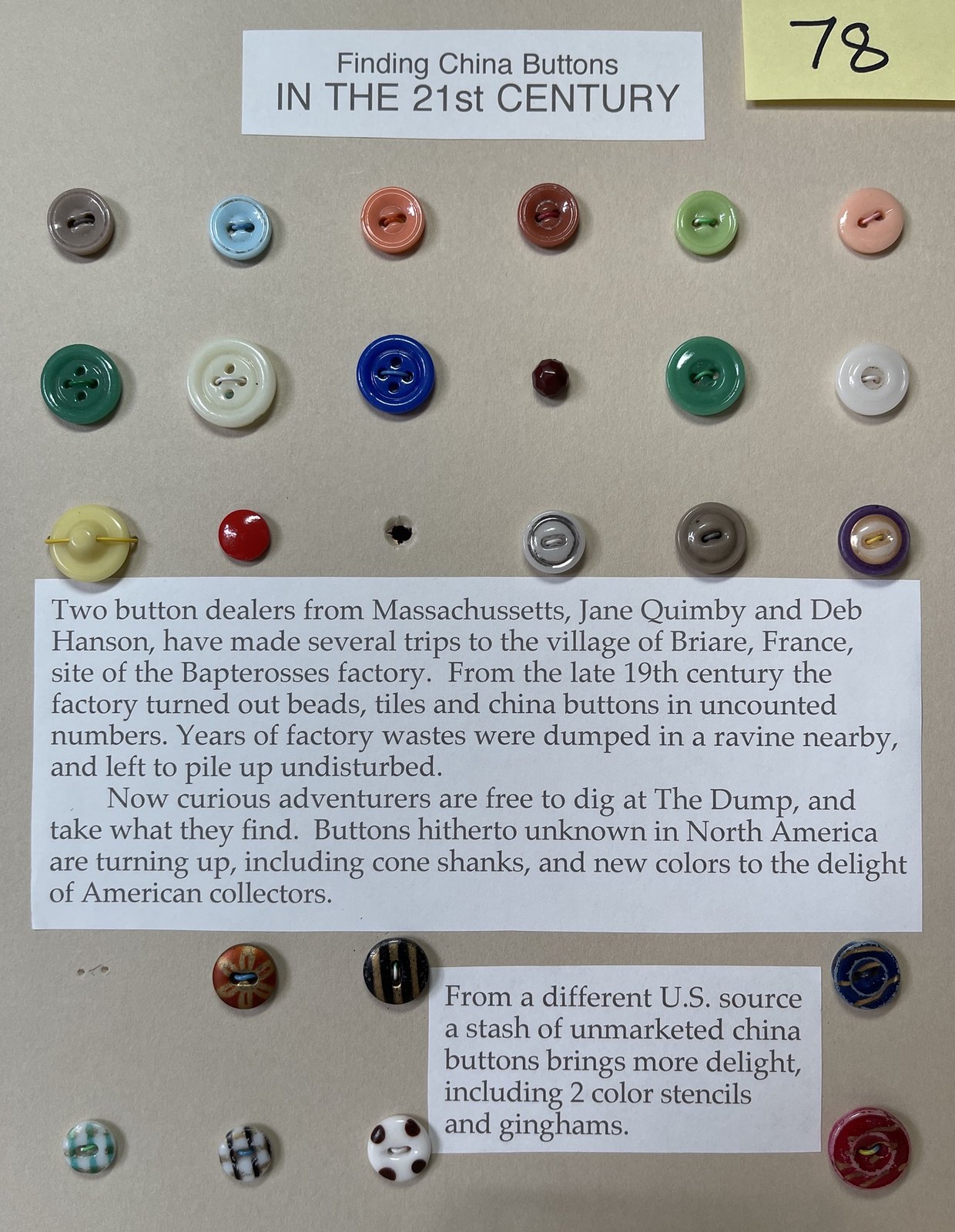The image showcases an extensive display of colorful China buttons scattered across a tan surface. The collection features buttons in a variety of colors such as yellow, black, white, tan, gray, light blue, orange, maroon, green, and blue, with some buttons exhibiting patterns like plaid and polka dots. Text at the top of the image reads, "Finding China Buttons in the 21st Century". The exhibit tells the story of two button dealers from Massachusetts, Jane Quimby and Deb Hansen, who have made several trips to the village of Brère, France. They explored the site of the Bacterius factory, which produced an immense number of beads, tiles, and china buttons from the late 19th century. The factory's waste, dumped into a nearby ravine, has remained undisturbed for years, now offering curious adventurers a chance to dig and unearth these historical buttons. The text details how buttons previously unknown in North America, including cone shanks and new colors, are now being discovered to the delight of American collectors. Additionally, a separate stash of unmarketed China buttons from a different U.S. source includes two-color stencils and gingham patterns, further intriguing button enthusiasts.